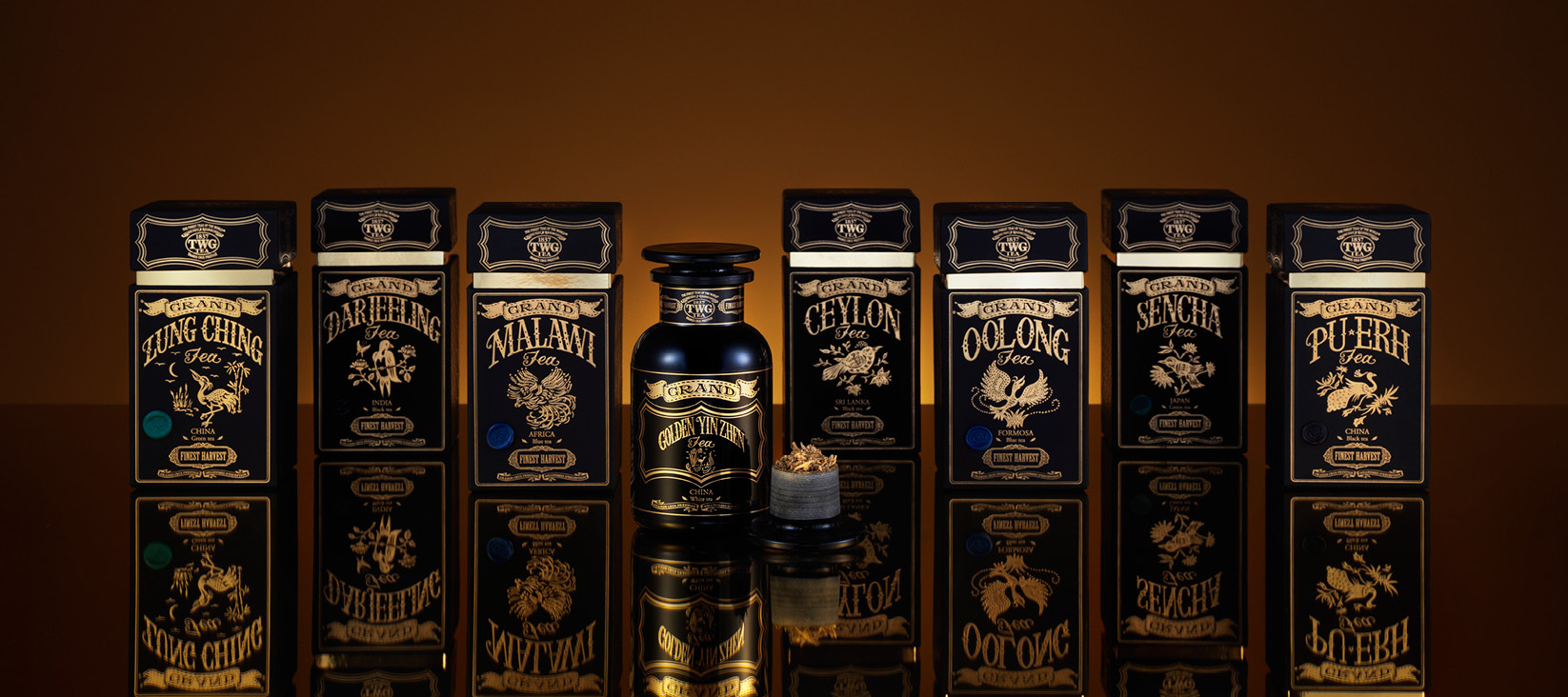This detailed color photograph, presented in a wide, landscape orientation, captures an elegant display of tea containers from the Grand brand (G-R-A-N-D) arranged on a highly reflective, brown surface. The primary subjects include seven dark blue to black boxes with distinctive gold logos, emblem, and writing. Starting from the left, the labels on the boxes read: Zung Ching, Darjeeling, Malawi, Ceylon, Oolong, Sencha, and Puer. 

In the center of this lineup is a matching dark blue jar adorned with similar gold decoration and a stopper lid, presumably containing tea as well. Notably, three of the boxes (the first, third, and fifth from the left) feature a blue circle on the bottom left corner. Additionally, a small glass container filled with what appears to be brown tea leaves is positioned beside the jar.

The reflective surface beneath the items captures their mirrored images, enhancing the high-end, upper-scale appearance of the products. The background reveals a gradation of brown, darker at the top and illuminated in the center, adding depth and focus to the composition. This photograph exemplifies a mix of photographic representationalism and realism, emphasizing product photography's detailed and luxurious style.